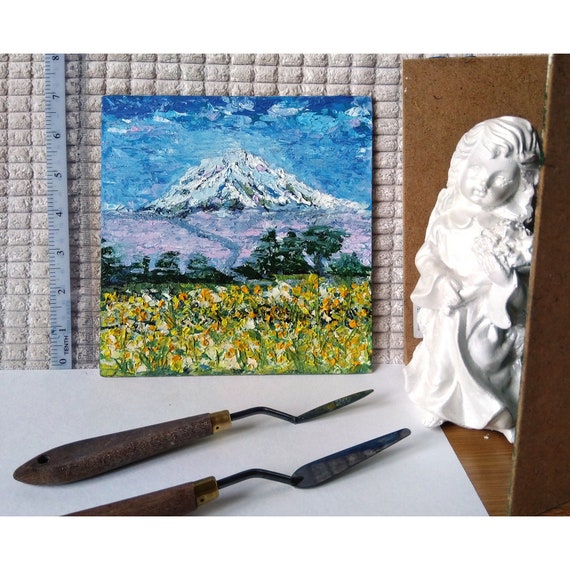A detailed image captures a scene set against a white tabletop or countertop with a light gray, checkerboard-patterned cloth on the back wall. To the right, there are pieces of brown cardboard or wood. Dominating the back wall is a square, vivid painting featuring a natural landscape: a snow-capped mountain with trees, yellow flowers, and a sky transitioning through blue, white, purple, green, yellow, and orange hues. Adjacent to this artwork is a ruler indicating the painting's dimensions, around 7 inches. Next to the painting stands an elegant white marble figurine of a woman with intricately carved details, including swooping hair and a long gown with sleeves. In the foreground, two palette knives with deep brown wooden handles rest on the white surface, seemingly out of place amidst the artistic tableau.